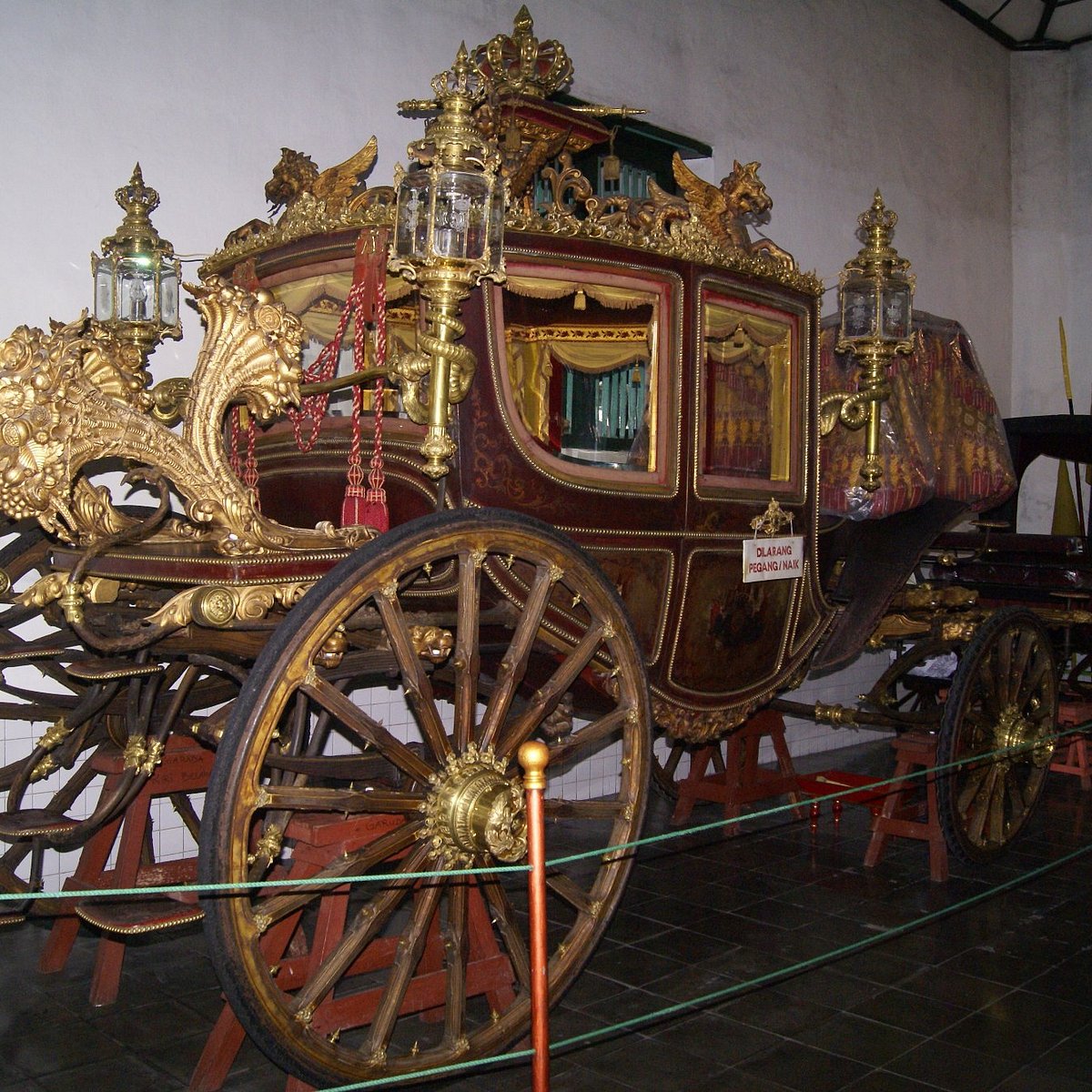The photograph, taken in a museum, captures an exquisitely ornate royal carriage displayed against a bright, white background wall and a brown square-tiled floor. The carriage is made of dark walnut wood embellished with intricate gilded gold decorations, including scrolls and designs. Four brass lanterns, mounted on snake-shaped arms, are positioned at each corner of the carriage, adding to its opulent appearance. The flat roof features gilded cherubs and intricately carved dragons with wings on each corner, alongside a central sculpture partially obscured from view. The carriage has large, elaborately designed wheels with golden hubs and multiple spokes, and it is elevated on small red sawhorse-like stands. The front showcases a rich array of details including a tasseled red rope and an upholstered flat seat. A prominent white and red sign, written in a foreign language, hangs from the carriage door. To prevent visitors from touching the display, there is a green rope fence tied to small wooden posts. The overall image is clear, brightly lit, and vividly colored, emphasizing the carriage's majestic craftsmanship.